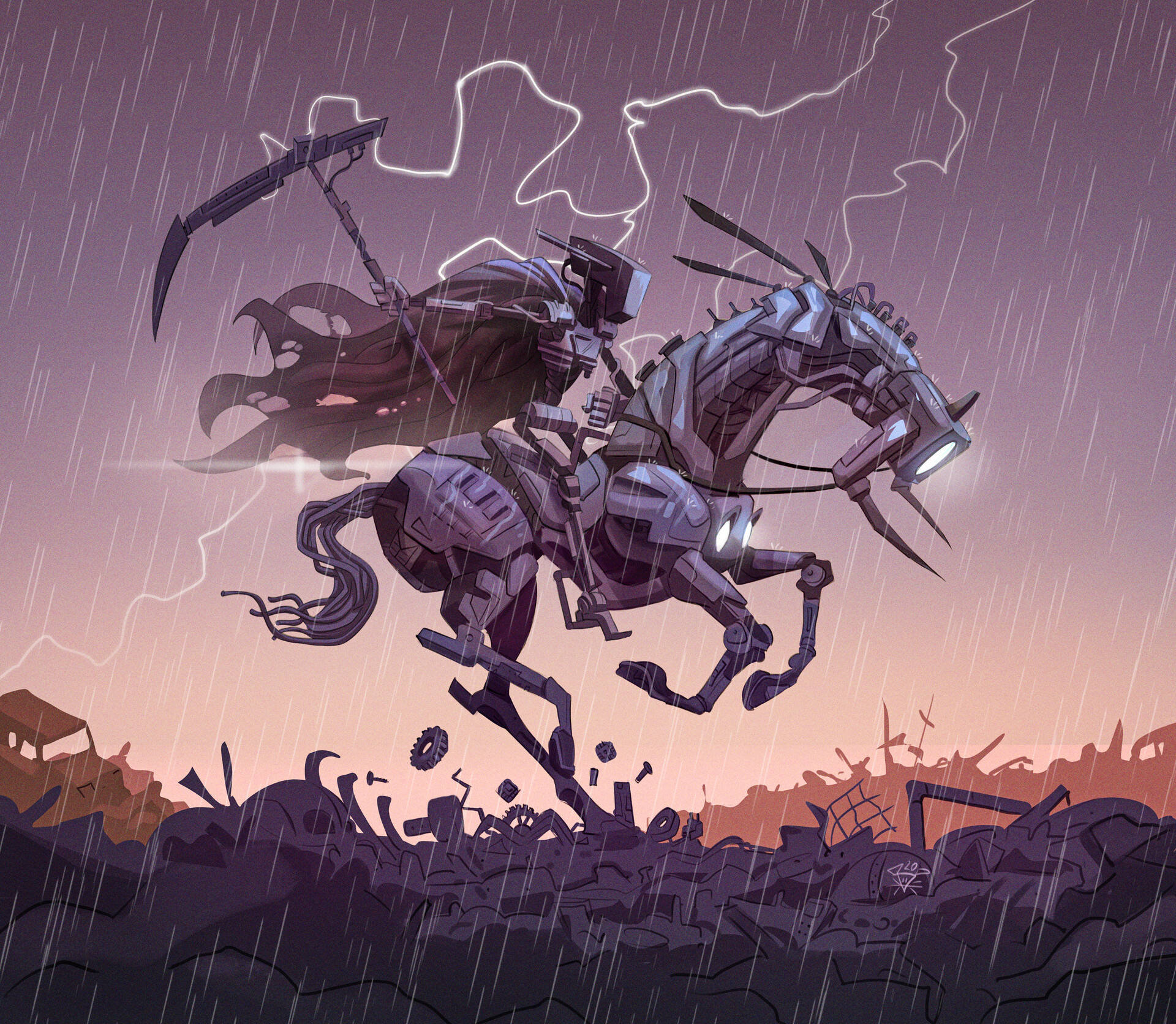The image is a detailed, rectangular drawing, roughly six inches wide and four to five inches high, depicting a scene filled with intricate mechanical elements and atmospheric conditions. Dominating the composition is a galloping mechanical horse, oriented from left to right. Its body is meticulously crafted from various shades of gray, featuring a headlight where its nose would be and two additional headlights on its chest, similar to car fog beams. Notably, the horse has tusk-like protrusions extending forward from either side of its head. 

On the horse's back rides a robot, characterized by the same metallic texture. This rider brandishes a large, segmented scythe and dons a tattered cape that flows dramatically behind it. The setting is a chaotic junkyard, with layers of debris beneath the horse's galloping hooves—gray at the base and transitioning to orange above. Various mechanical components like screws and nails appear to be flying up from the ground, indicating motion and speed.

The sky above mirrors the mechanical, eerie feel of the ground below. It transitions from a light peach color at the horizon to a mauve purple as it ascends, with rain seemingly falling and a prominent lightning bolt streaking down. A faint silhouette of a vehicle looms in the background, adding to the scene's dystopian atmosphere. The entire artwork combines desaturated hues and vibrant details, creating a compelling juxtaposition of mechanical and natural elements.